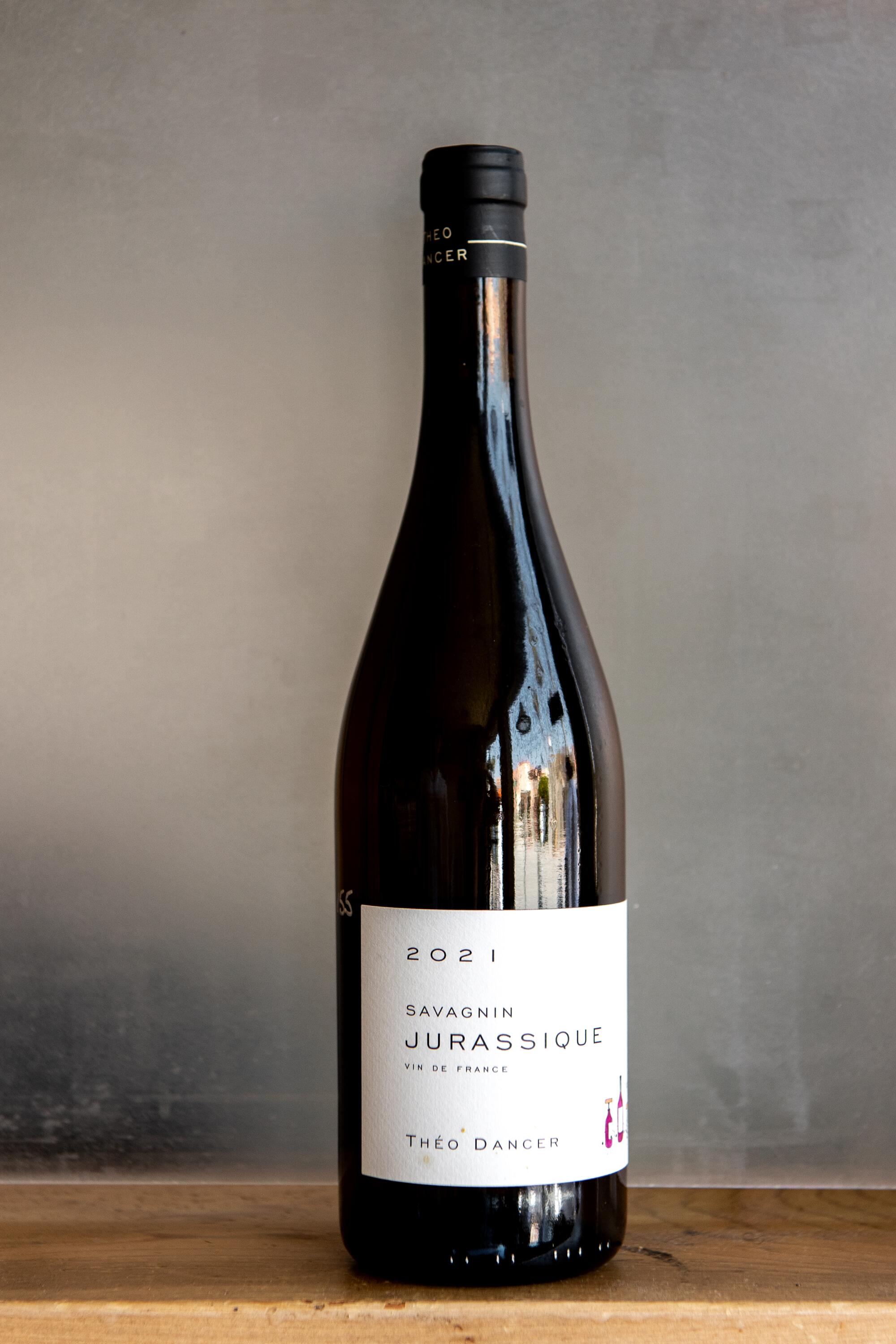The image features a tall wine bottle prominently displayed on a wooden counter with a grey, chalkboard-like background. The bottle has a dark, almost black hue with a black cap. The white label on the bottle displays "2021" and "Sauvignon Jurassic" in black font, accompanied by the mention "Vin de France" and the name "Theo Dancer" at the bottom. There is a small red image, possibly depicting wine bottles or glasses, located near the bottom right of the label. The picture captures a reflection on the bottle's right side, which appears to include indistinct figures. This close-up photograph offers a detailed and appealing presentation of the bottle.